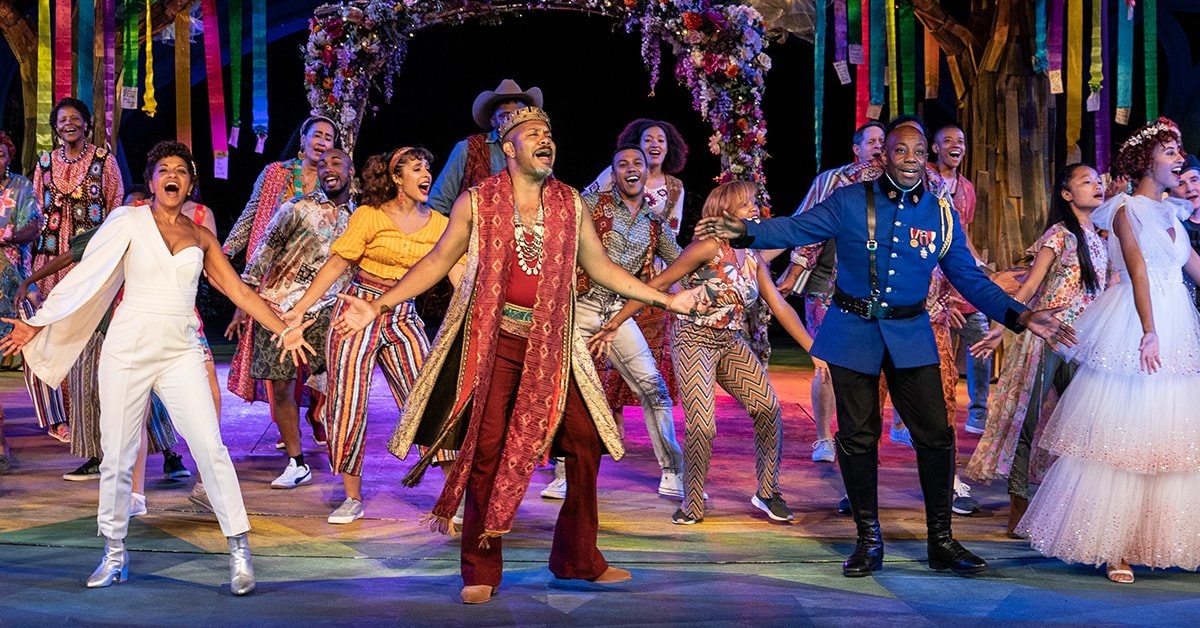This vibrant photograph captures an exuberant musical performance on a colorful stage adorned with rainbow hues. In the foreground, an Indian man, donning a sleeveless red and gold diamond-patterned vest and a crown, stands prominently with his arms outstretched, leading the cast in song. To his left stands an African American woman in a one-sleeved stark white outfit, while another African American woman wears a colorful brown vest. A black man in traditional Indian attire and an Indian woman in a yellow vest with striped yellow, red, and white pants add to the diversity of costumes. The right side of the stage features an African American man dressed as a police officer, his blue uniform adorned with medals. Additional cast members, dressed in a mix of colorful and traditional attire, stand in the background. The stage floor is a burst of colors, with reds, blues, purples, yellows, and greens, mirroring the vibrant streamers hanging from the rafters. An arch made of various flowers forms a stunning backdrop, enhancing the theatrical and joyous atmosphere of this indoor performance. The lighting from above illuminates the scene, emphasizing the performers' wide-legged stances and open-mouthed expressions as they sing in harmony, creating a sense of unity and celebration.